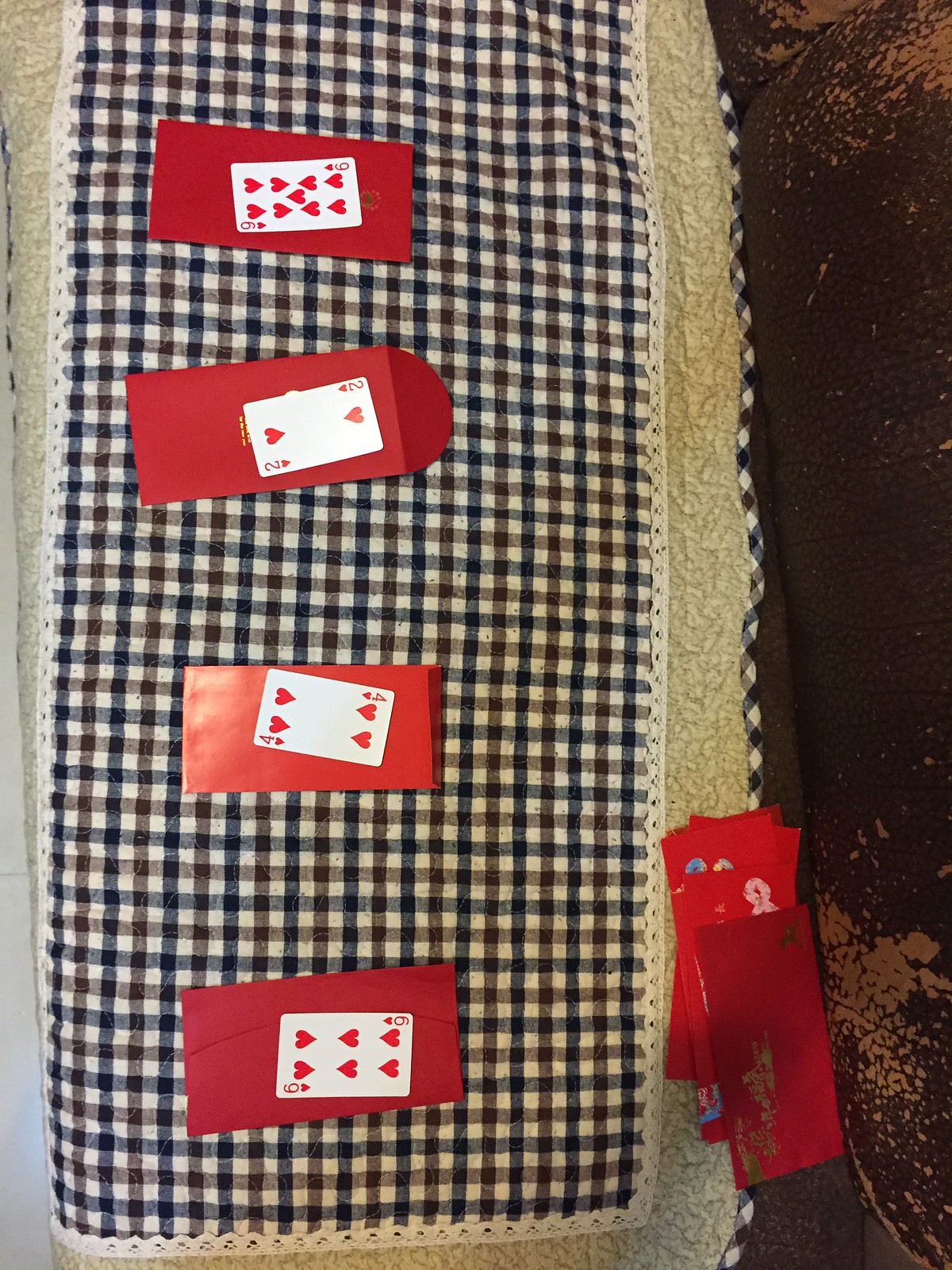In the foreground of the image, a collection of playing cards is displayed, all showcasing their suit sides—hearts, diamonds, clubs, and spades—none of them revealing their decorative backs. Each card is delicately placed on top of a red envelope. Some of these envelopes are positioned to show the flap, while others reveal the opposite side. 

Behind this arrangement of cards and envelopes, there is a patterned background featuring a grid of rows and columns. The colors used in this grid are predominantly black, white, and shades of gray, with intricate borders resembling lace. This background fabric has a textured appearance, hinting at a woven or carpet-like material. The borders are adorned with intersecting lines that run diagonally from corner to corner, creating a dynamic contrast.

In the lower right corner of the image, there is a small stack of unused red envelopes. Adjacent to this stack, another surface is visible, possibly made of leather or imitation leather. This surface might be part of a chair base or another object. The lower section of the image hints at a cloth underneath the cards, possibly placed within a booth seating area. The booth seat, which appears to be upholstered in leather or a similar material, extends to the right, suggesting a cozy and intimate setting.